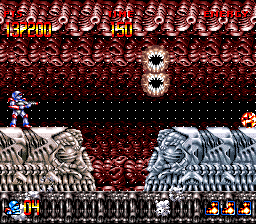The image is a screenshot of a vintage 2D side-scrolling video game with pixelated graphics, portraying a surreal, intestine-like background filled with red and maroon tentacle-like structures. Prominent in the scene is a figure in a blue and red suit standing on a tan, skeletal train on the left side, while a mirrored silver skeletal train is positioned to the right. Above these trains, two menacing mouths with white, spiky teeth are visible, and the entire scene is dotted with small white points forming a grid.

On the left side, there is a small character, while a fireball floats on the right side. The game interface shows the player’s head icon at the bottom left, followed by the number '04'. Spaced out along this bottom interface are symbols of a grayed-out fireball and three orange fireballs encased in blue borders. The top section includes red and orange text indicating 'points', a score of '150', and the word 'energy', enhancing the retro gaming aesthetic. Figures with teeth are stacked vertically toward the middle left, further adding to the quirky and eerie environment.